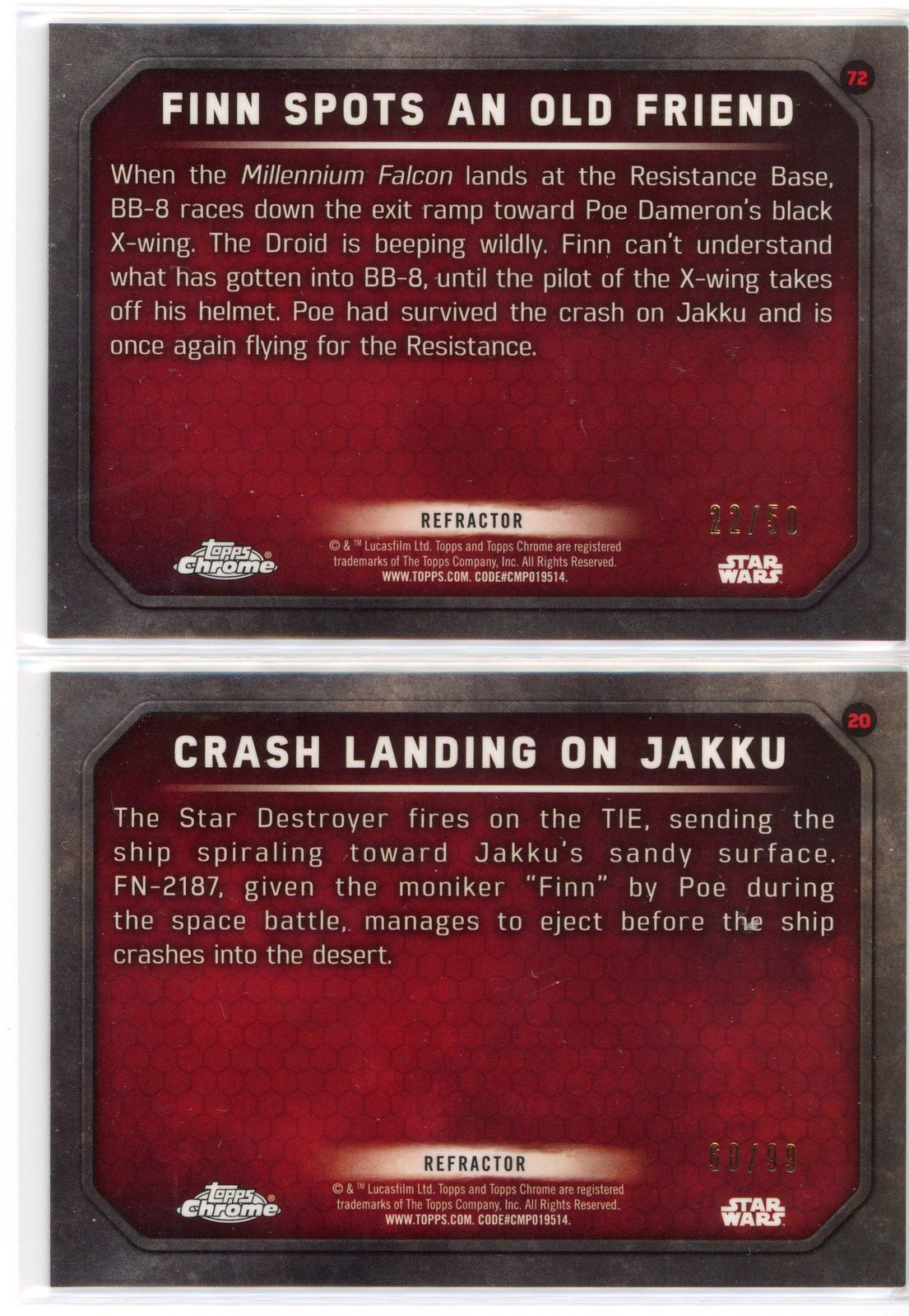This image features the back side of two Star Wars Topps Chrome Refractor trading cards, each serially numbered in gold at the bottom right (the top card is 22 out of 50 and the bottom card is 60 out of 99). Both cards share a burgundy background with a dark gray border and white text. 

The top card is titled "Finn Spots an Old Friend" and is numbered 72 in the set. The detailed description reads: "When the Millennium Falcon lands at the Resistance Base, BB-8 races down the exit ramp toward Poe Dameron's black X-wing. The droid is beeping wildly. Finn can't understand what has gotten into BB-8 until the pilot of the X-wing takes off his helmet. Poe has survived the crash on Jakku and is once again flying for the Resistance."

The bottom card is titled "Crash Landing on Jakku" and is numbered 20 in the set. Its description states: "As the Star Destroyer fires on the TIE, the ship spirals toward Jakku's sandy surface. FN-2187, given the moniker Finn by Poe during the space battle, manages to eject before the ship crashes into the desert."

Both cards feature the Topps Chrome and Star Wars logos, as well as a "Refractor" label and associated copyrights at the bottom of each card.